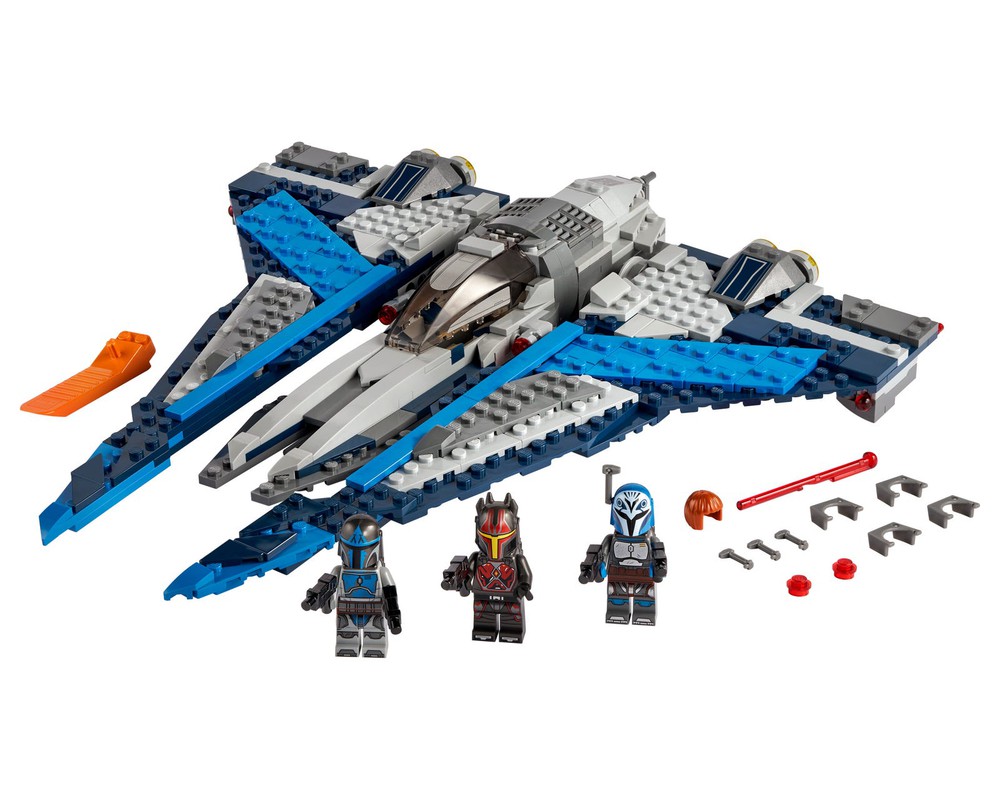In this detailed image of a Lego set, we see a striking Star Wars or Mandalorian-themed scene set against a white background. Dominating the photo is a meticulously constructed starfighter, with a predominantly gray body accented by light blue lines within its wings and dark blue edges. The starfighter features a cockpit in the center and jet propulsion mechanisms at the rear, and includes a distinctive orange ramp-shaped piece to the left side. 

In front of the starfighter stand three detailed Lego characters resembling Mandalorians, equipped with futuristic black phaser guns. The character on the left is outfitted in light blue, gray, and black, while the one in the middle sports a dark gray, red, and yellow ensemble. The character on the right is adorned in light blue, white, and gray. Scattered around these figures are additional accessory pieces, including a lightsaber constructible and other colorful components, adding to the detailed and imaginative display of this Lego set.